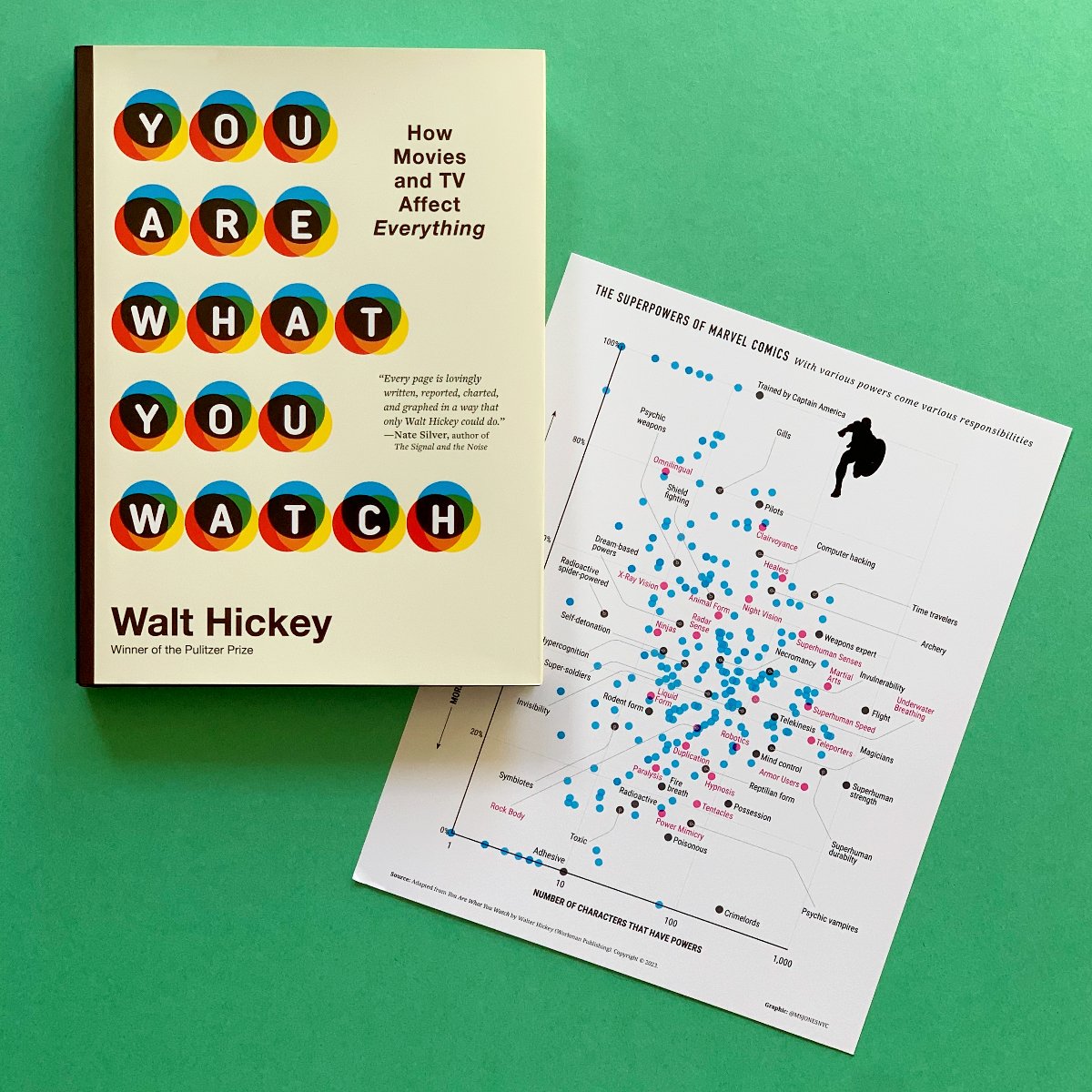Set against a mint-greenish background, this real-life photograph captures a book and a sheet of computer paper slightly overlapped and positioned near the lower right. The book, showcased in the upper left corner, features a title in bold, colorful circles that merge into black centers, spelling out "You Are What You Watch" in uppercase white letters. Underneath the title, the subtitle reads, "How Movies and TV Affect Everything" in black text. Credit goes to Walt Hickey, prominently noted at the bottom as a "Winner of the Pulitzer Prize." Additionally, a small quoted recommendation from Nate Silver, author of "The Signal and the Noise," praises the book's detailed and graphical reporting.

To the right of the book lies a white sheet titled, "The Super Powers of Marvel Comics: With Great Powers Come Great Responsibilities." The document, which resembles a chart, is somewhat obscured by the book but displays numerous multicolored dots plotted on a graph. The Y-axis is marked from 0 to 1000, named "Number of Characters that Have Powers," while the other axis is hidden. The sheet also features a silhouetted image of Captain America running towards the viewer, adding a dynamic element to the scene.